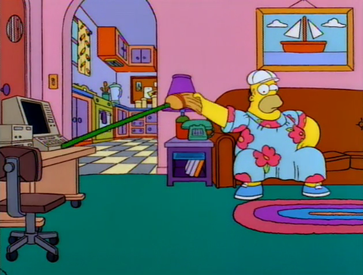In this still frame from the television show "The Simpsons," the iconic living room is depicted with meticulous detail. On the left-hand side of the image, an arched doorway leads into a kitchen distinguished by its blue and orange cabinets and adorned with yellow curtains on the window. In the foreground, an antique-style computer sits on a table at the far left side of the living room, accompanied by a wheeled office chair. To the top-right corner of the scene, a painting of a red sailboat navigating blue waters under white clouds hang in a brown frame. Below this painting, the family's brown couch is prominently placed, serving as the seating for Homer Simpson. Homer, dressed in a whimsical outfit featuring a white golf hat, a blue and red-flowered muumuu, and blue shoes, is innovatively using a broom’s handle to push a button on the computer from across the room. The floor of the living room is an intriguing blue-green hue and a vibrant rug with concentric circles of pink, blue, and purple adds a splash of color to the space. This scene captures the eccentric and endearing charm characteristic of "The Simpsons."